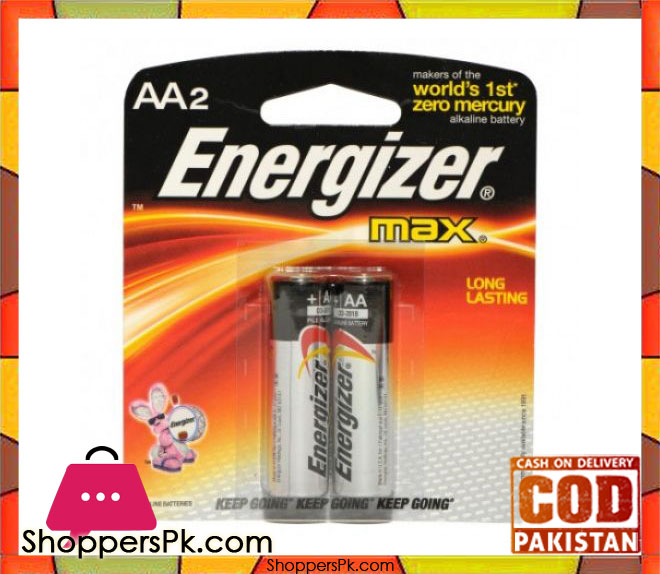The image features a vibrant geometric background composed of intersecting shapes outlined in black, filled with a blend of orange, green, and brown hues. Central to the image is a large white square with a photograph of an Energizer Max battery pack prominently displayed. The packaging has a sleek design: the top section is black while the bottom part transitions through orange, yellow, and white colors.

In the upper left-hand corner of the battery pack, the text "AA 2" is printed in white capital letters. On the right side of the packaging, a yellow label proclaims, "World's First Zero Mercury." A standard cutout at the top of the packaging, designed for store displays, is also visible.

Dominating the center of the packaging, the brand name "Energizer" is written in large, bold white letters outlined in black. Just below this, the word "Max" appears in yellow, also outlined in black. At the bottom center of the packaging, two AA batteries, which have black tops and silver bottoms, are showcased; each battery features the iconic Energizer logo in their recognizable red and yellow colors.

To the left of the batteries, the cheerful pink Energizer bunny, equipped with sunglasses and a bass drum, is prominently displayed. In the bottom left corner of the image, a small pink purse with three central dots can be seen, accompanied by the text "shopperspk.com" in black lettering.

In the lower right corner, a distinct square contains the phrase "cash on delivery" at the top, followed by large, uppercase letters "COD," and the word "Pakistan" beneath them.